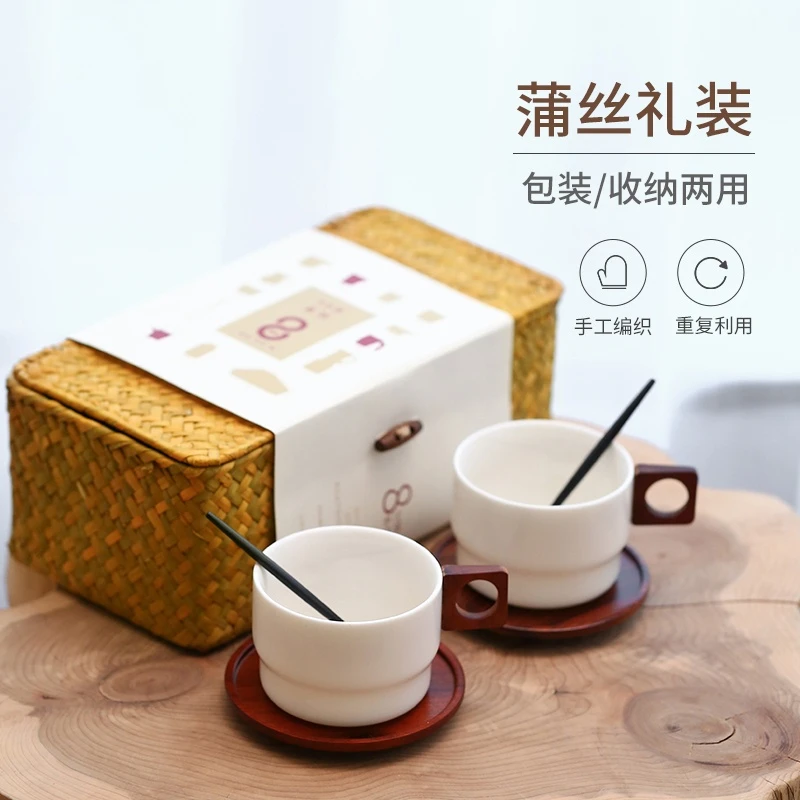This is a Japanese advertising poster set against a blue, blurred background. At the center of the composition is a cut log of a tree, displaying its growth rings and patterns, serving as a natural and rustic platform. Positioned on this tree trunk platform is a beautiful bamboo woven basket, wrapped with a white label featuring various shades of maroon and cream.

In front of the basket are two white ceramic cups, each equipped with a distinctive wooden handle featuring a square hole for easy grip. Each cup contains a black chopstick-like stirring stick. The layout is meticulously arranged, showcasing the articles in an aesthetically pleasing manner.

In the top right corner of the poster, there are Chinese symbols or letters accompanied by a pair of circular icons. One icon features a kitchen mitt, and the other represents a fast forward or rewind symbol, both adorned with additional Chinese text underneath. This rich blend of traditional and modern elements paired with the clean design invites viewers to explore the melding of craftsmanship and utility.